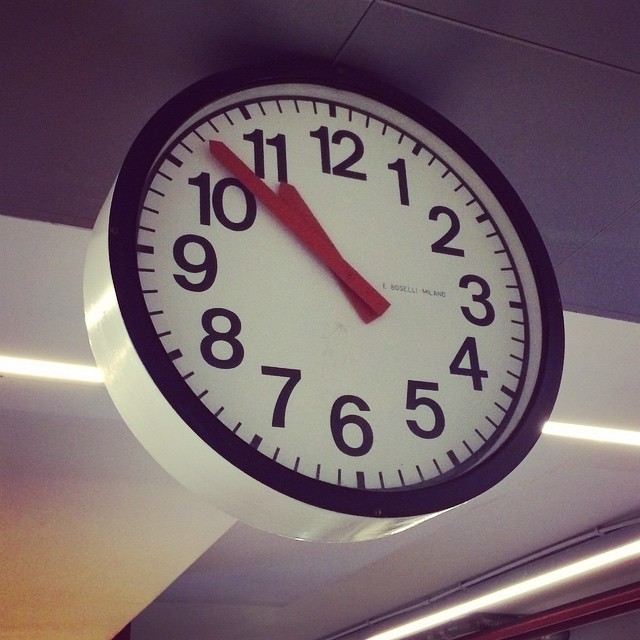This detailed photograph captures a round, ceiling-mounted clock with a darker body color and a white clock face. The clock features black numbers and black dashes marking the minutes, with the number "3" accompanied by black text. Two red hands indicate the time. The ceiling surrounding the clock includes a strip of white lighting and a white wire-like object running nearby. Additionally, another strip light is visible in the frame, accompanied by a touch of red trim in the corner. Light reflections shimmer off the clock's body, adding depth to the image.